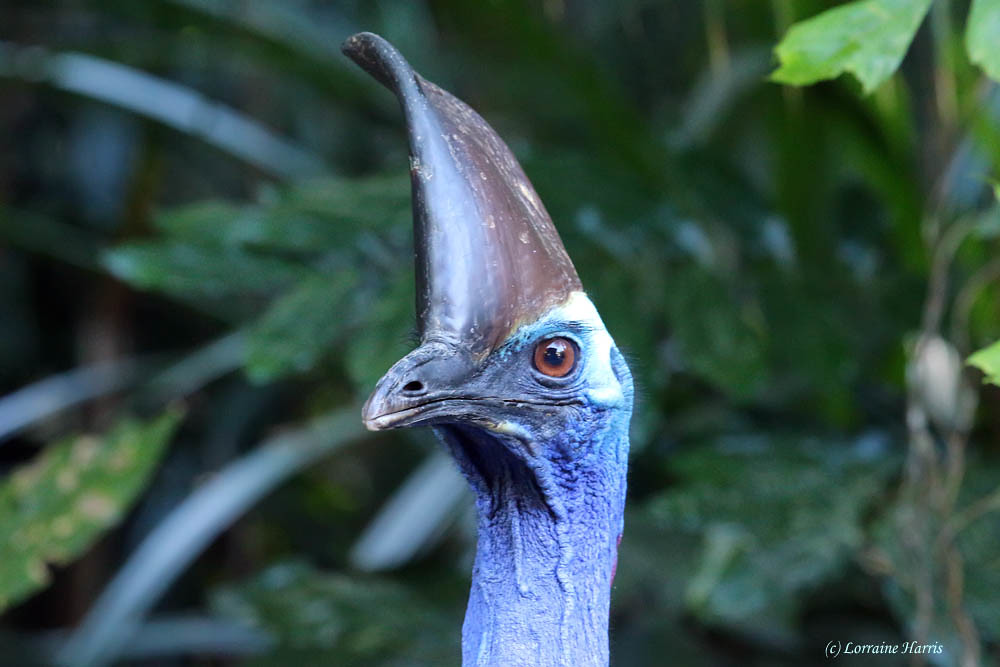This is an image of a cassowary, captured in a horizontally oriented, rectangular frame. The photograph is a close-up headshot of the bird from the neck up, focusing on its distinctive features. The cassowary’s head and facial skin display varying hues of blue, with a patch of white towards the back of its wrinkly, featherless neck. Its beak is a subtle blend of grayish-black, and it has a large, prominent brown eye. Towering above its head is a tall, thin horn, characterized by dark brown and black colors, slightly curved and marked with signs of wear. The background of the image consists of blurred, green foliage, likely comprised of large leaves, which accentuates the vibrancy of the bird’s colors. The focus remains centrally on the cassowary’s head, with a copyright symbol and the name "Lorraine Harris" in white text located at the lower right corner of the picture, indicating the photographer.